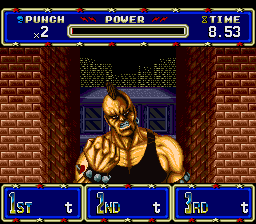The image depicts a vintage fighting video game, likely from the 1980s, showcasing a muscular man with a light beige skin tone and a brown mohawk standing in the center. The man, with a blue mouth and brown eyes, sports notable features such as blue circle ring earrings, a tattoo of a red heart with an arrow on his right shoulder, and black bands with blue dots on his upper arms. He wears a sleeveless dark brown t-shirt and has his right fist raised in front of his chest, head slightly tilted to his right.

In the background, there are two large brick pillars framing the character and a blue building, possibly high-rises with yellow-lit windows, adding depth to the scene. The upper portion of the screen features a prominent blue banner, trimmed in bright blue and gold, displaying text elements: "Punch X2" and a nearly depleted power bar. To the right, next to an hourglass icon, the time reads 8:53. The bottom of the screen showcases UI elements in blue boxes with gold trim, stating "first T," "second T," and "third T," mirroring the design of the top banner.